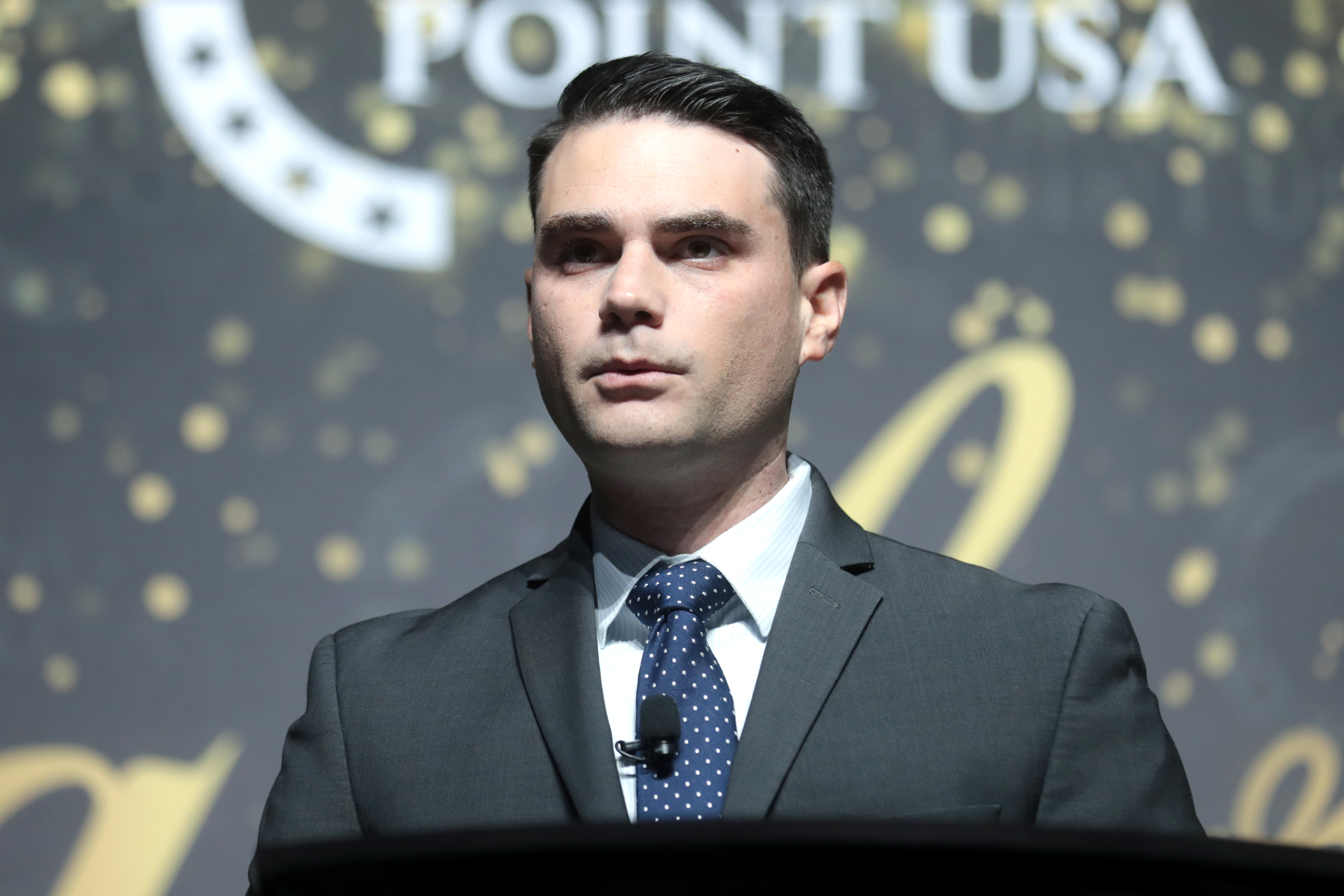In this indoor photographic setting, a young man, probably in his late 20s or 30s, is captured wearing a sharp gray suit paired with a white dress shirt and a blue tie adorned with white polka dots. He has short, slicked-back black hair, bushy eyebrows, and is clean-shaven. A small microphone is attached to his shirt. The man is looking slightly away from the camera with his lips pursed, giving a composed and attentive expression. 

In the background, a gray backdrop features a distinct design with yellow stars, and prominently displays the text "Point USA" in white. Surrounding the word "Point" is a curved band with small black stars. There are also sections of cursive letters visible in the lower left-hand and right-hand corners, although not fully readable, potentially forming letters such as an "a" or an "L". The overall setting suggests a professional or special event atmosphere, with intricate details lending to a sophisticated scene.